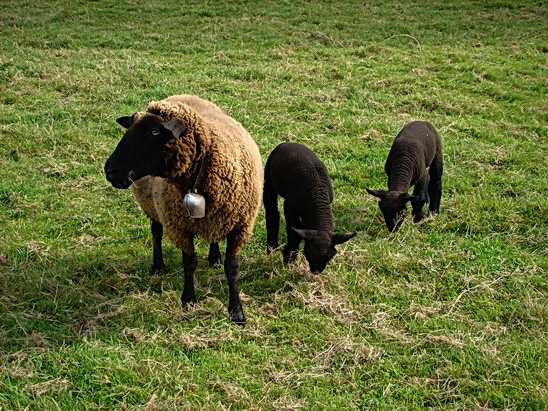In this clear daylight photograph, we see a green grassy field interspersed with patches of dried grass and hay. Dominating the frame is a large adult sheep, situated just left of center, with a brown woolly coat, black face, and black legs. Around its neck hangs a silver bell. The adult sheep is looking towards the left side of the image, exuding a protective demeanor over its two young lambs, which are positioned to its right. The lambs are entirely black, with short hair and their heads lowered as they graze on the lush grass. One lamb is oriented to the right, while the other faces the center left. The bright sunlight enhances the colors and casts shadows to the left of each animal, highlighting the serene agricultural setting.